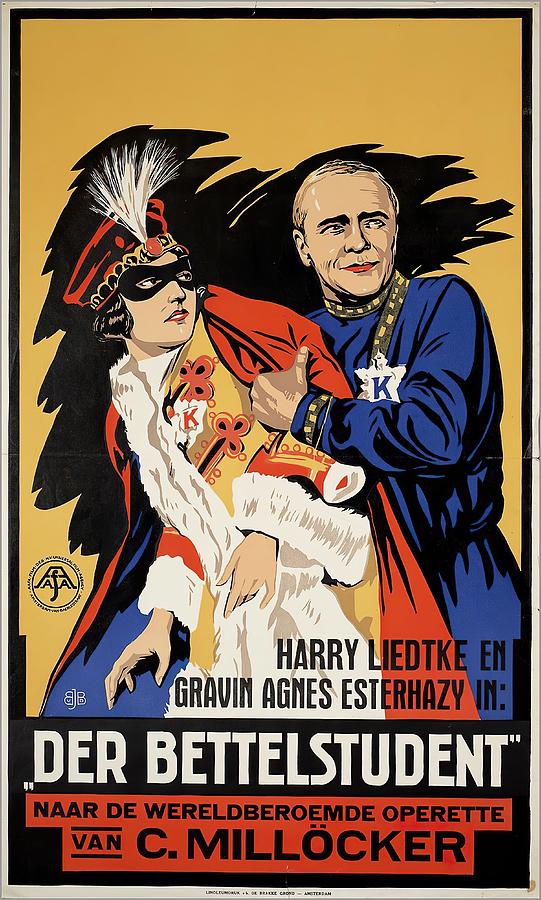The image is a vividly colored poster, likely from the 1940s or 1950s, advertising a movie or a play. It features a thin gray border followed by a thin black border, thicker at the bottom. The backdrop is predominantly yellow with some elements in black. Two central figures dominate the poster: 

On the left, there is a woman dressed in an elaborate long red robe adorned with white fur on the cuffs and running down the front from her neck area. She wears a red hat with gold embellishments and a plume of feathers and has a black mask covering her eyes. 

To the right, there is a man in a long blue robe with gray hair. He wears decorative jewelry, including a necklace with a star symbol featuring the letter "K." 

The text on the poster reads "Harry Liedtke, Gavin Agnew, and Esther Hazy," with additional text indicating "Der Bettelstudent" and other indistinct phrases, further suggesting it's an advertisement for a theatrical or cinematic production.